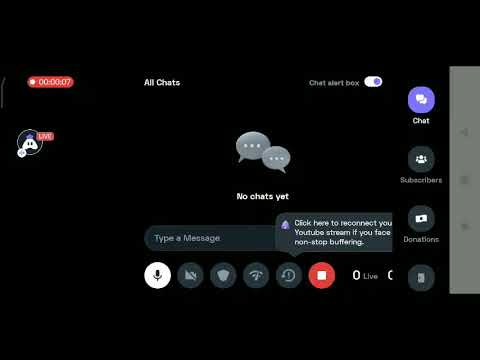The image is a screenshot from a chat application, likely from a YouTube stream, characterized by a predominantly black background. On the right-hand side, there is a vertical array of four circular icons. The top circle is purple, featuring a white speech bubble icon with the label 'Chat' underneath. Below it, a gray circle contains an icon of multiple figures, labeled 'Subscribers.' The third circle, also gray, displays a dollar bill icon labeled 'Donations.' The lowest circle shows a door icon but isn't labeled.

In the top left corner, a red oval contains the number '0000007', indicating a time stamp of seven seconds with a 'LIVE' badge nearby. Slightly to the right, the text 'All Chats' is visible, with a chat alert box toggle next to it. 

Centrally placed on the screen are two speech bubbles with the message 'No chats yet' beneath them, and directly under this, a text field prompts users to 'Type a message.' Adjacent to the message field, there is a notification message saying, 'Click here to reconnect your YouTube stream if you face non-stop buffering.'

At the bottom of the screen, there's a series of circular control icons. The first icon is white with a small microphone inside. Next, dark gray circles host a camera, a shield, a Wi-Fi indicator, a refresh symbol, and finally, a red circle with a white square, likely representing a stop button.